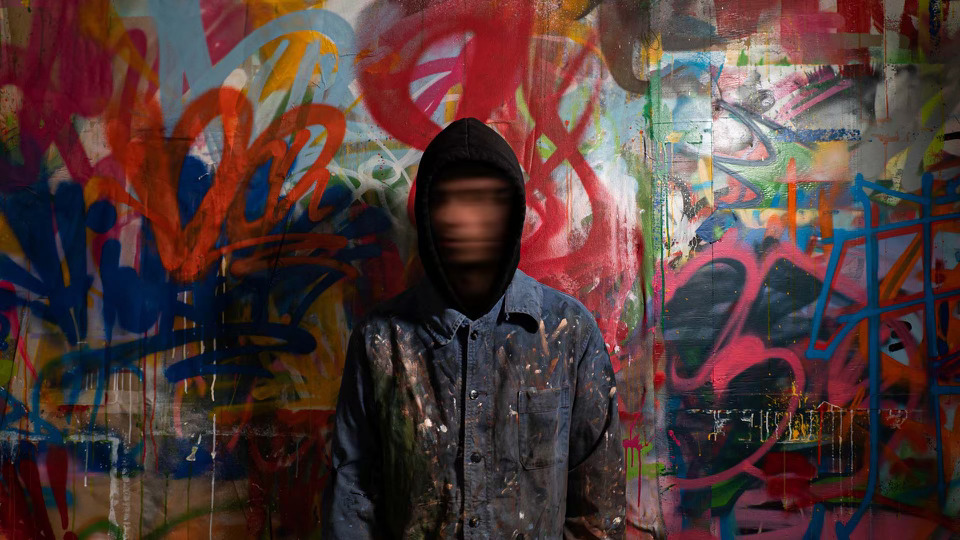This photograph, professionally taken with a realistic aesthetic, features a horizontally oriented image dominated by an expansive graffiti-covered wall. The wall's surface, possibly composed of metal or brick, is densely adorned with a chaotic fusion of graffiti art in a vibrant array of colors: red, blue, yellow, pink, orange, gray, white, green, dark pink, and black. The sheer volume of overlapping symbols, squiggles, and indecipherable text renders the individual contributions indistinguishable.

Centrally positioned against this vivid backdrop is a man, whose attire suggests he might be the graffiti artist. He wears a distressed denim button-up shirt, heavily smeared with paint, and a black hoodie that covers his head. Paint notably stains the left sleeve of his long-sleeved shirt, reinforcing his potential ties to the artwork behind him. The man's head is captured mid-motion, shaking rapidly from side to side, resulting in a blur that obscures his facial features; this effect could be either a deliberate photographic technique or computer enhancement, adding a sense of dynamism to the image.

The composition suggests a carefully crafted piece of art, possibly serving as the artist's promotional photograph, showcasing both the individual's enigmatic identity and his colorful, collective creation on the wall.